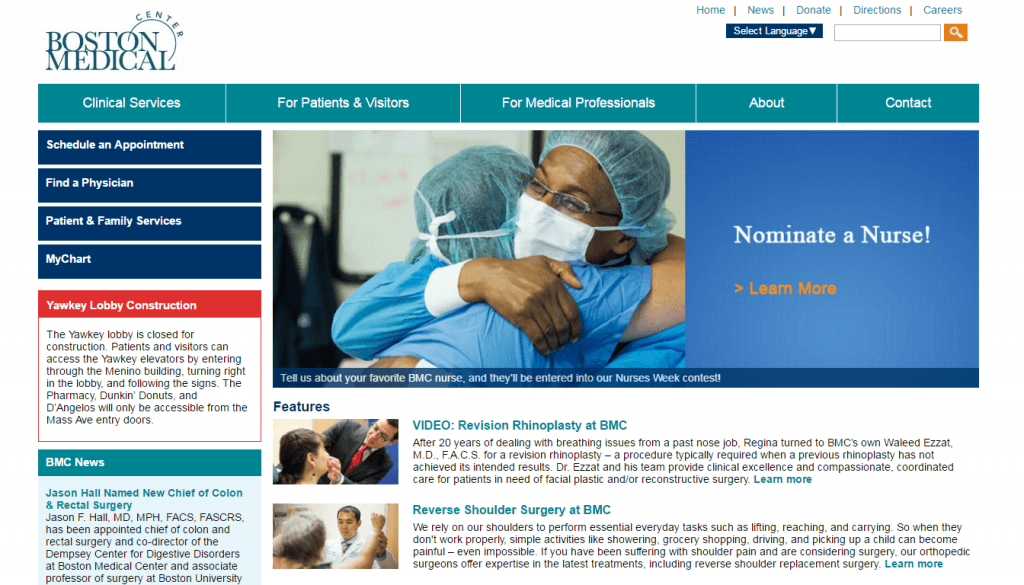The web page of Boston Medical Center offers a comprehensive overview of services and information for various audiences. The top section of the page features navigation links for Home, News, Donate, Directions, Careers, language selection, and a search box.

**Main Headline and Highlighted Features:**
Prominently displayed is a headline encouraging visitors to "Nominate a Nurse." Users are invited to share stories about their favorite BMC nurse, who will be entered into a Nurses Week contest. This section includes a call-to-action button to "Learn More."

**Left Side Navigation:**
On the left side of the page, there are several navigation buttons, including:
- Schedule an Appointment
- Find a Physician
- Patient and Family Services
- MyChart
- Yawkey Lobby Construction Notice

**Construction Advisory:**
There is an important notice highlighted about the Yawkey lobby being closed for construction. Visitors are advised to access the Yawkey elevators through the Menino building by turning right in the lobby and following the signs. Additionally, essential facilities like the Pharmacy, Dunkin’ Donuts, and D’Angelo’s remain accessible via the Mass Ave entry doors.

**Additional Content:**
The website also covers promotional content, news updates, videos, and information on medical procedures such as rhinoplasty and reverse shoulder surgery.

**Overall Description:**
The Boston Medical Center web page effectively combines informational content with practical guidance for patients, visitors, and medical professionals. The layout supports easy navigation and provides timely updates on services and facilities, ensuring visitors have access to all necessary information in an organized manner.